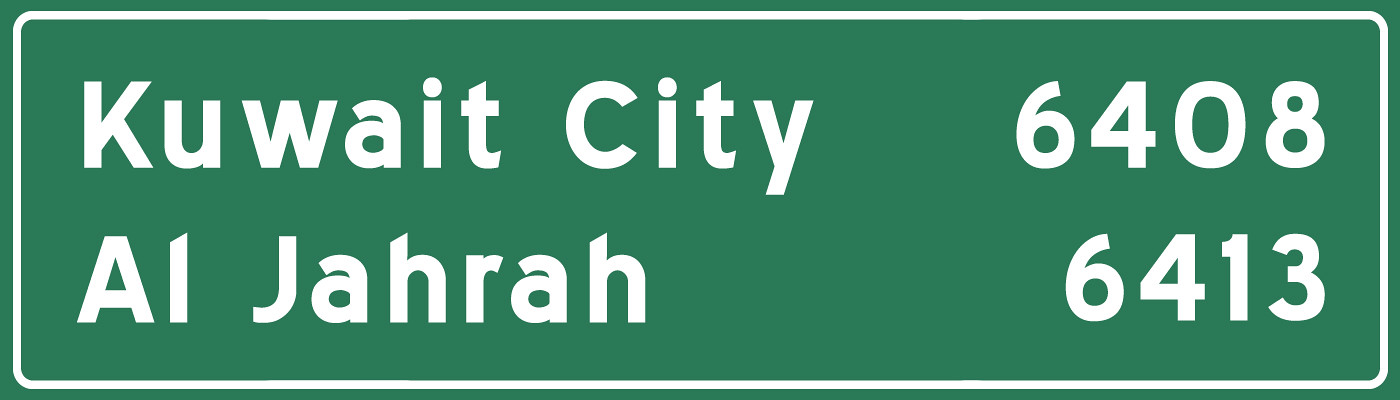A rectangular road sign prominently displaying essential directional information. The sign features a green background with a white border sandwiched between two green sections. At the top, the sign reads "KUWAIT CITY" in clear, uppercase letters, followed by the number "6408." Below this, "AL JAHRAH" is written in a similar fashion, accompanied by the number "6413." The sign's design and color scheme are meant to ensure high visibility and readability for drivers seeking directions to these locations.